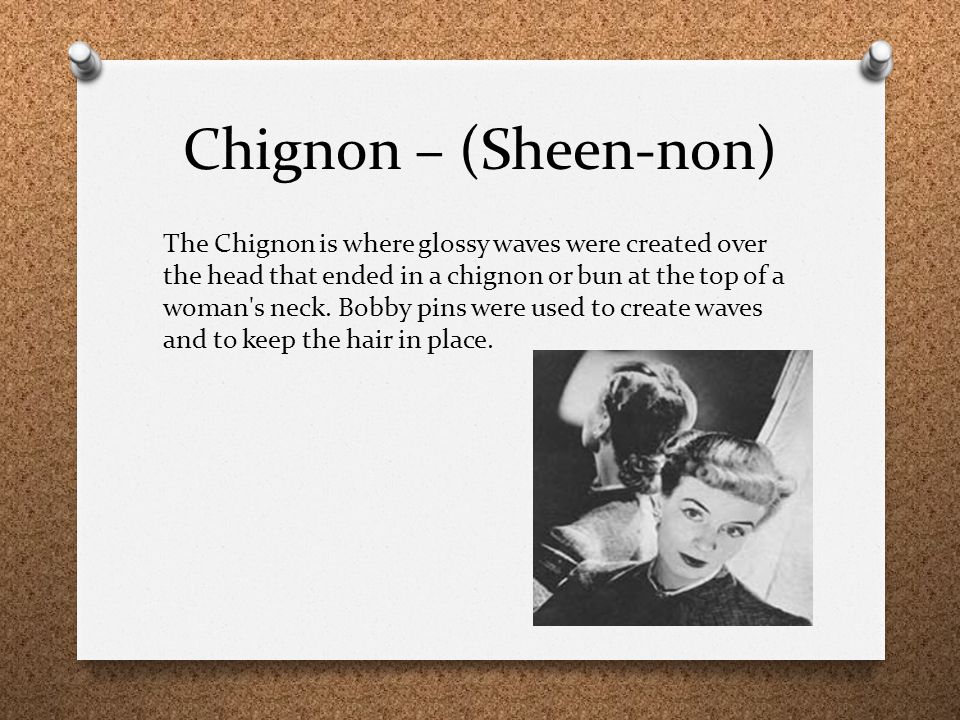The image depicts a digitally-created poster pinned to a bulletin board made of cork material. The poster, modeled on standard printer paper, is secured at the top corners with two silver tacks. The title on the poster reads "Chignon" followed by a pronunciation guide in parentheses: (SHEEN-non). Below the title, a paragraph explains that a chignon involves creating glossy waves over the head that culminate in a bun at the top of a woman's neck, held in place by bobby pins. Positioned in the lower right corner of the poster is a black-and-white photograph of a woman with a 1950s-style hairdo. She faces the camera with a mirror behind her, reflecting the back of her head and right shoulder, showcasing the chignon hairstyle.